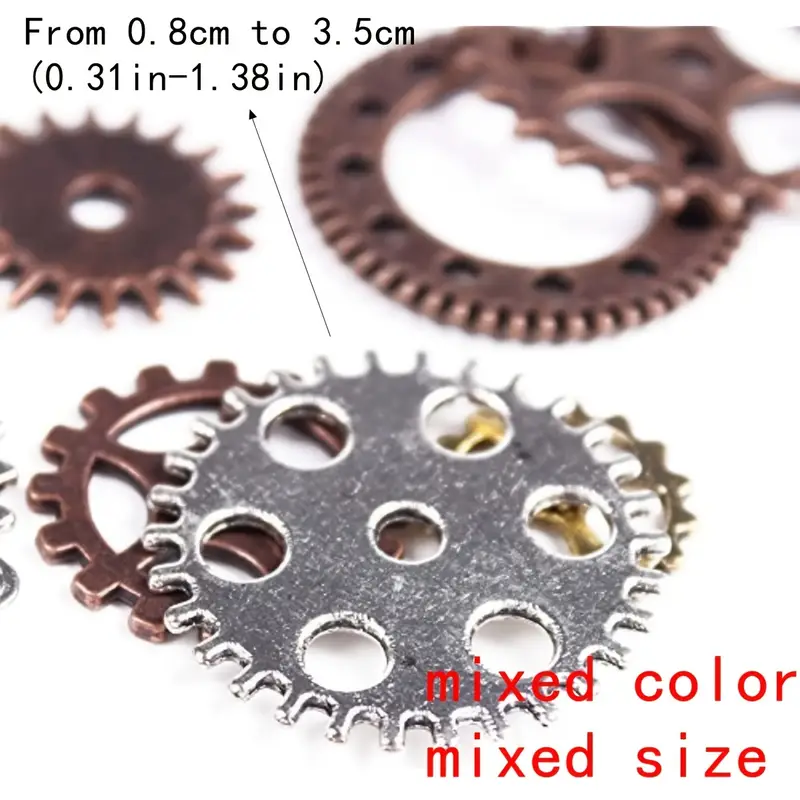This is a detailed color diagram depicting an assortment of differently shaped gears, resembling bicycle sprockets, made from various metals such as brass, bronze, and stainless steel. The size range from 0.8 cm to 3.5 cm (0.31 inch to 1.38 inch) is clearly marked in black text at the top left of the image. At the bottom right, in red text, it states "mixed color, mixed size." The gears vary not only in size but also in design and color: some are silver, others bronze, and a few even appear golden. Notable examples include a prominent silver gear in the foreground with six outer circles and a central circle, a brown gear with jagged, spiky edges, and another brown gear featuring notched edges and black spots around a large central opening. Additionally, there's a brownish gear on the lower left with rounded square shapes around its perimeter.